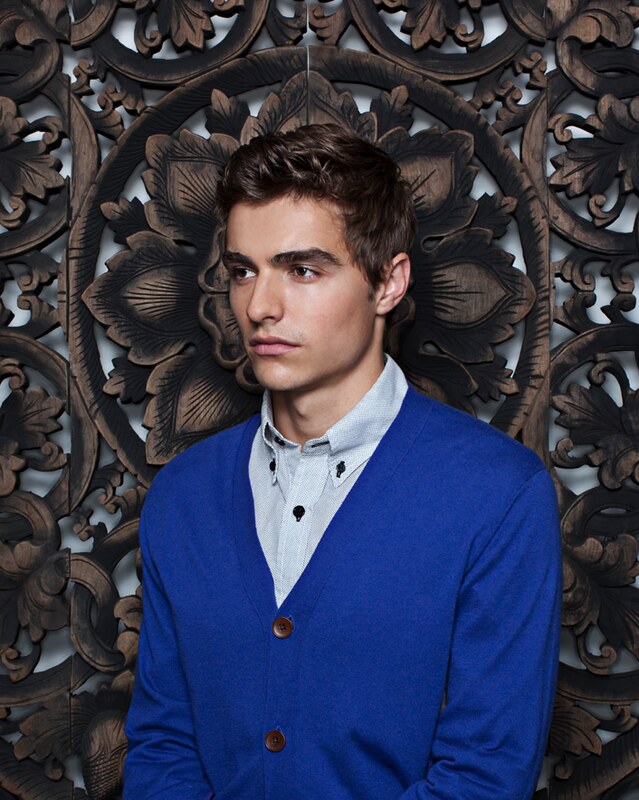The image is a color photograph in portrait orientation, showcasing actor Dave Franco. He has short dark brown hair and very thick eyebrows, and he is posing with a serious, contemplative expression on his face. Franco is dressed in a bright blue cardigan with brown buttons, under which he wears a light blue formal shirt with black buttons. He is pictured from the top of his head to near his elbows and is turned to his side at a 45-degree angle, slightly looking downward, allowing his profile to be prominently featured.

The background features an intricate, ornate carved wooden mural with a floral pattern against a white wall. The centerpiece of the mural, a large blossoming flower, is positioned directly behind Franco's head, complemented by smaller flowers and elegant scrollwork encircling it. The use of flash has cast shadows of this detailed wooden sculpture onto the white background, further emphasizing its sophisticated craftsmanship. The overall style of the photograph is highly realistic, capturing finely detailed elements of both the subject and the background.